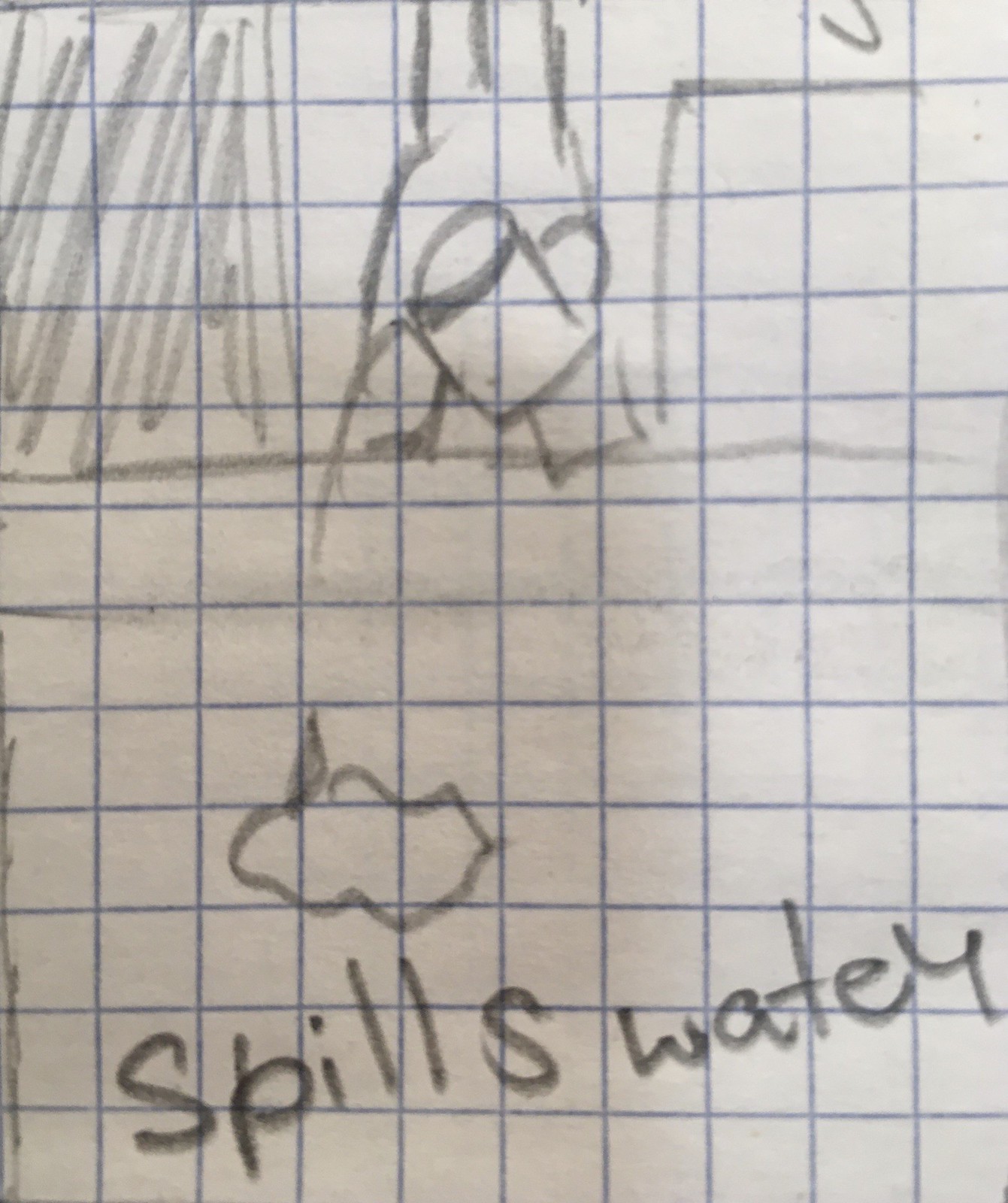A hand-drawn pencil sketch on a piece of blue-lined graph paper captures a scene involving a liquid spill. At the bottom of the paper, the phrase "Spills Wadi" is inscribed, possibly implying "spills water." Just above this, a wavy-edged circle-like object is depicted, which might represent the resulting puddle of the spilled liquid. 

At the top of the drawing, a horizontal line spans the page. Above this line, scribbled pencil shading fills the left side, suggesting an unfinished or abstract background. In the center, a detailed sketch of a pitcher or a can with a lid and a handle is shown. The pitcher is tilted, pouring liquid, presumably water, downward. Near the pitcher, there appears to be an indication of a person holding it, although the figure is indistinct and difficult to discern. The intricacy of the liquid flow and the careful attention to the graph lines add a unique texture to the composition.